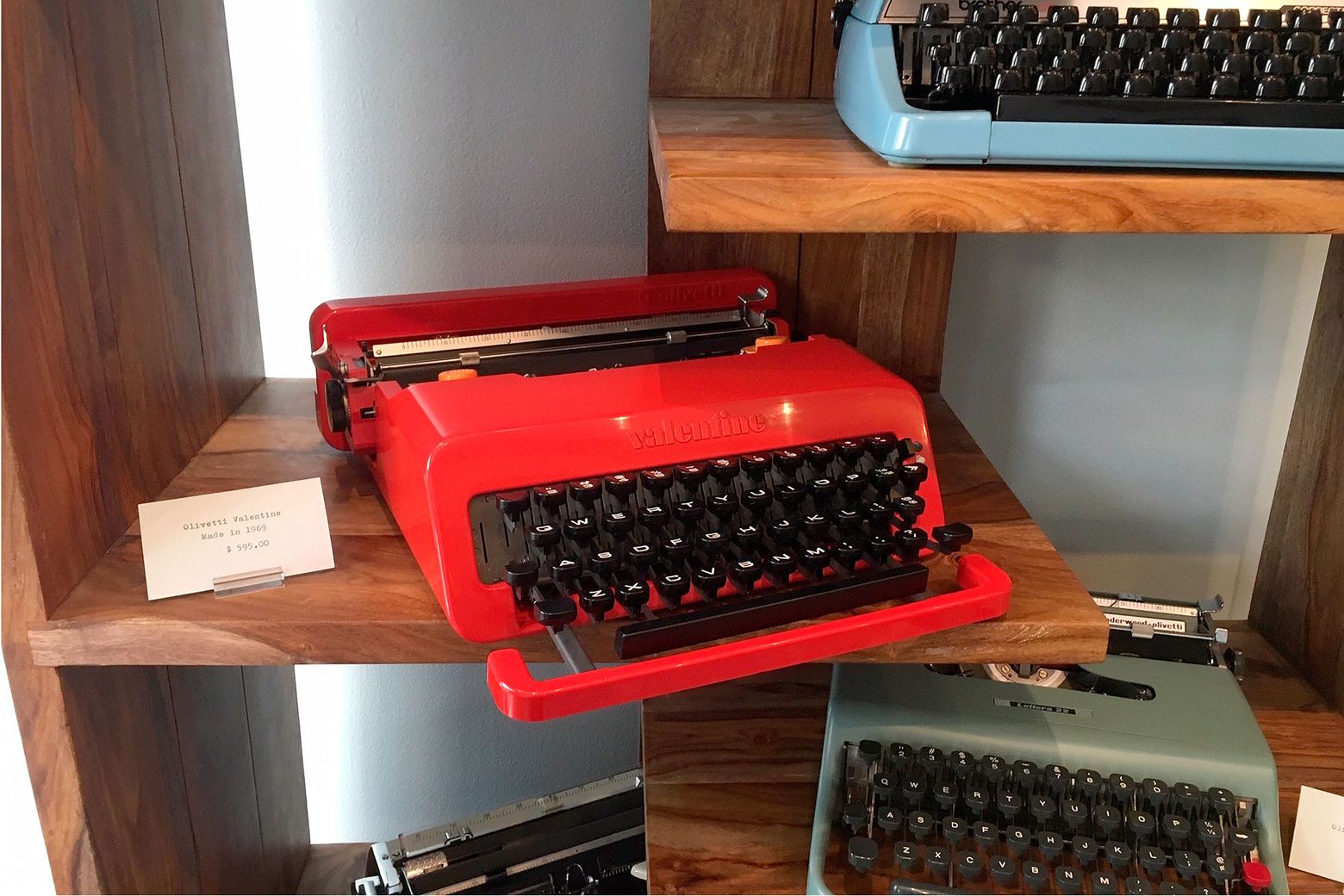The image showcases a series of layered, brown shelves, each supporting vintage typewriters in a display-like setting, reminiscent of a museum exhibit. At the top right, the bottom section of a blue typewriter is visible, featuring black keys arranged in a QWERTY layout. Below this, on the next shelf, there is a red typewriter labeled "Valentine," accompanied by a display card reading, "A La Vista Valentine, Code ID 1962, $595." Further down to the right, a light green typewriter with less distinct black keys is positioned, also flanked by a small, unreadable card. Positioned on the bottom left, another typewriter, this one presumably silver, completes the display. Each typewriter appears well-maintained and shiny, suggesting they are in good condition despite their vintage status.